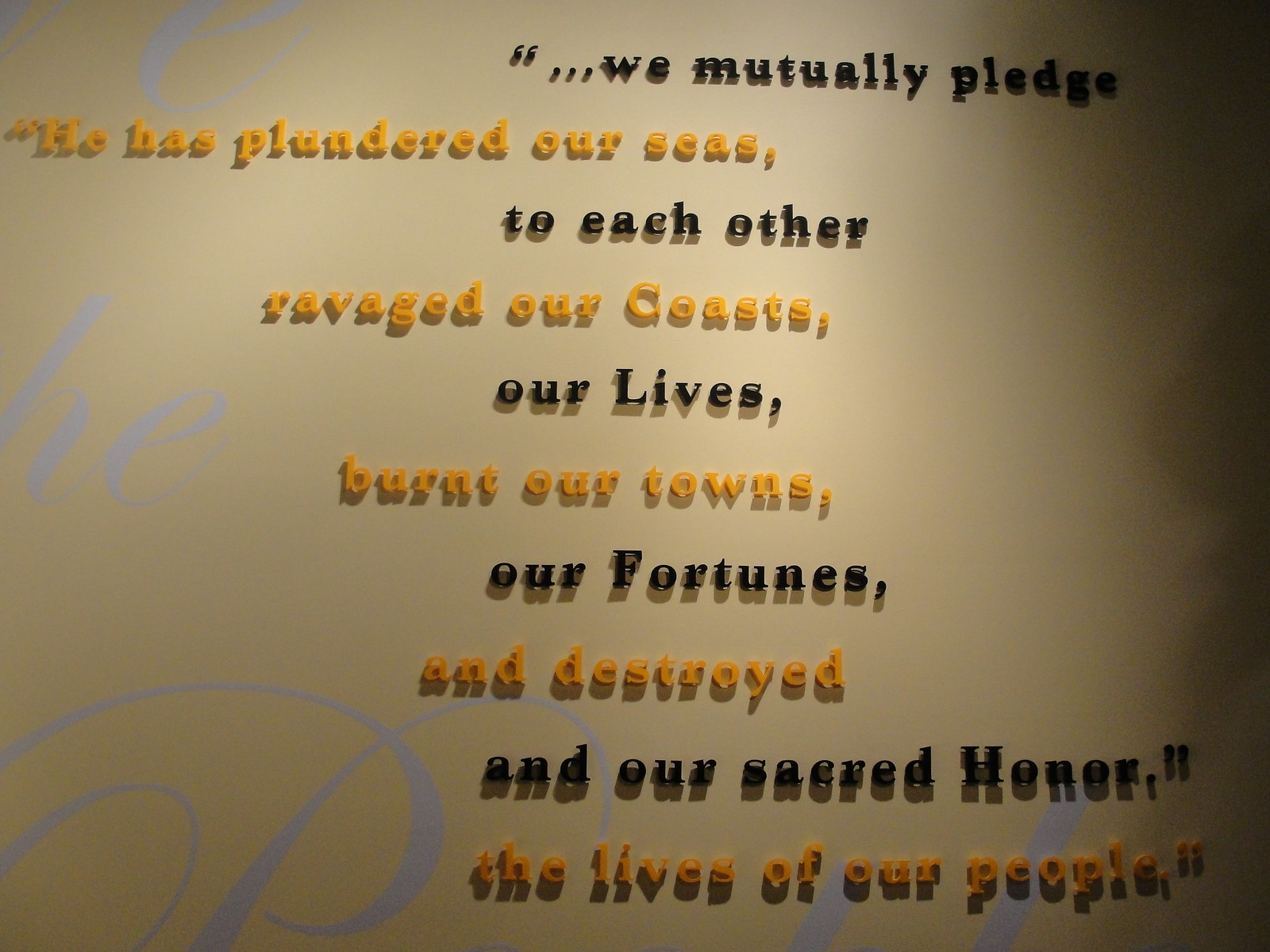The photograph captures an intricately designed piece of text, mounted on a wall with a light brown to yellow-gold gradient background that darkens towards the right. The text is presented in alternating lines of black and orange, creating a visually striking effect. The lines in black read, "We mutually pledge to each other our lives, our fortunes, and our sacred honor," while the lines in orange state, "He has plundered our seas, ravaged our coasts, burnt our towns, and destroyed the lives of our people." Although the text is shaded for emphasis, some cursive blue writing is faintly visible in the background, with partial letters such as 'H' and 'E' discernible. The entire inscription, framed with quotation marks, appears to juxtapose a pledge of unity against a series of grievances, making the message both poignant and evocative.